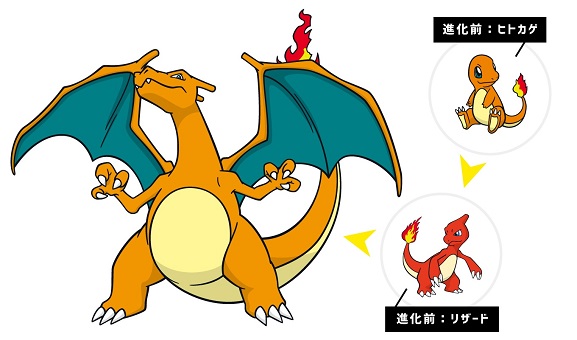The image displays a detailed cartoon sequence of the Pokémon evolution from Charmander to Charmeleon to Charizard. The characters are prominently labeled in Japanese with additional annotations next to each Pokémon. The largest and most prominent figure is Charizard, a yellow-gold dragon with green wings outlined in orange and a flaming tail, standing on its right legs with visible sharp fangs and claws. To Charizard’s right, two smaller images depict the earlier evolutionary stages: Charmander, a small orange dragon with a cream-colored belly and a flaming tail; and Charmeleon, red with a cream-colored belly and also a flaming tail. These smaller images are enclosed in bubbles with arrows indicating the evolutionary progression from Charmander to Charmeleon to Charizard. The text includes a mix of Japanese kanji and additional characters, potentially hiragana, distinctly set apart to provide specificity. The clear visual and textual elements together effectively convey the progression of this iconic Pokémon evolution.